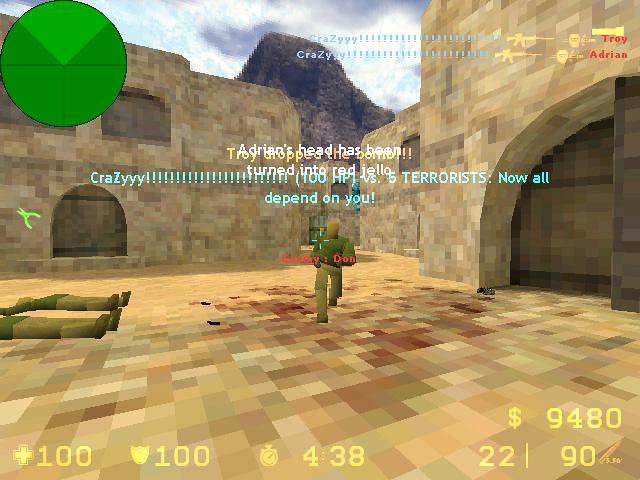The image, a pixelated screenshot resembling Minecraft, showcases a video game scene with a tannish, block-textured ground marked by reddish spots. A character with a green shirt and tannish pants is running while looking to the left. Two similar figures lie on the ground, presumably defeated. A large green circle with a V-shaped lighter green segment in the upper left corner serves as an overhead map, divided into quadrants by vertical and horizontal lines.

In the top right corner, red text displays the names "Troy" and "Adrian," accompanied by yellow gun icons and blue text exclaiming "crazy!!!" Below these names, yellow indicators read "100, 100, 438," signifying health, shield, and a clock time, respectively. The bottom right corner shows a monetary value of "$9480," and an ammunition count labeled "22/90." Additional text at the bottom of the screen reads, "Adrian's head has been turned into red jello. Terrorists now all depend on you," indicating a crucial status update in the game. The enemy mentioned is "Dan."